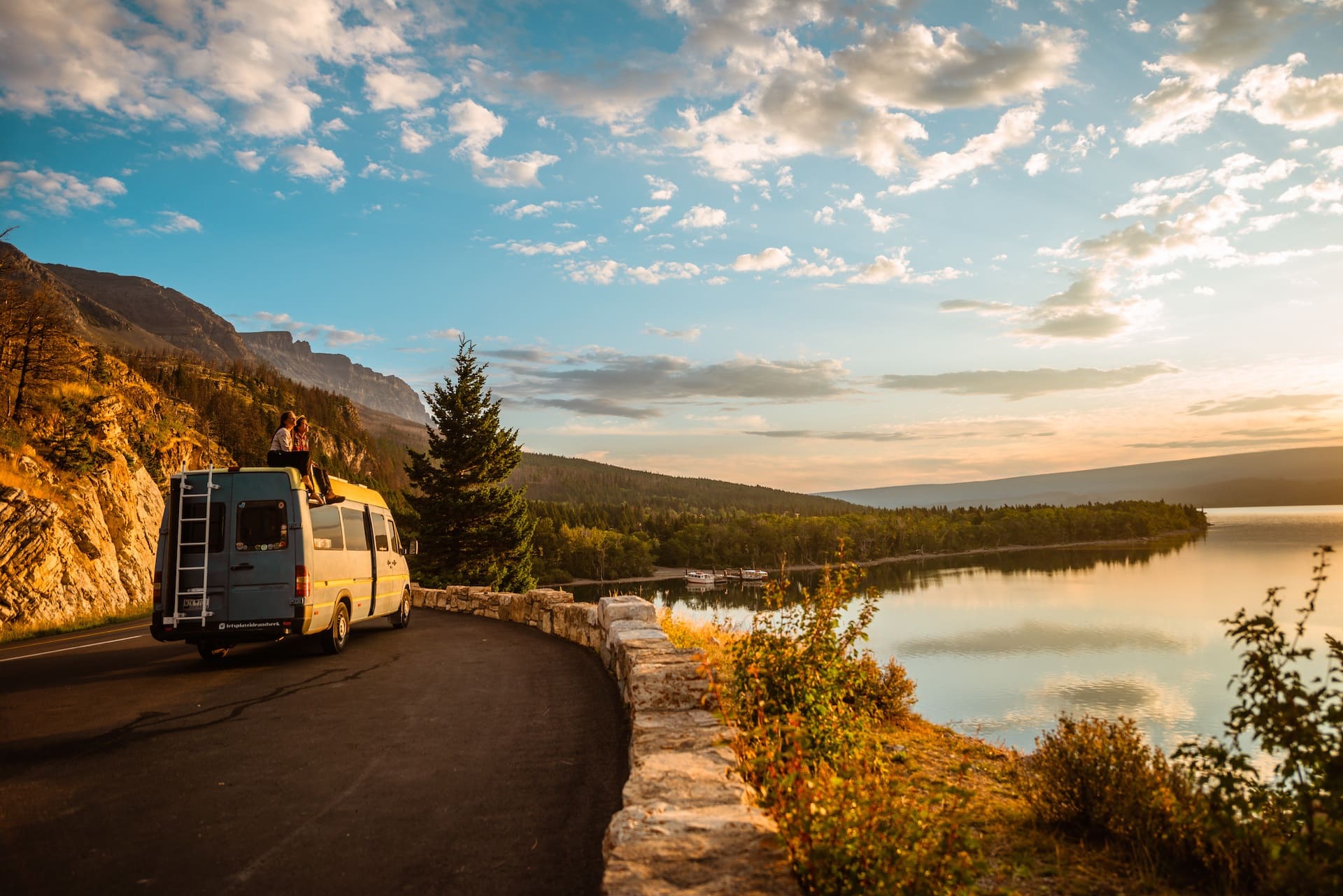This image captures a serene and picturesque moment where a camper van is parked at a scenic lookout spot high on a hillside. The road, narrow and winding, is flanked by a rocky mountain adorned with grasses on the left and a modest stone wall or rocks, likely serving as a safety barrier, on the right. The van, possibly blue or white, features a ladder at the back, adding to its rugged, exploratory charm. Two females are seen sitting atop the van, basking in the tranquility of the moment as they gaze out over a nearby lake that glistens under the setting sun. The sky is a beautiful gradient of blue and orange hues, merging into a cloudy backdrop. In the distance, pine trees dot the rocky mountain slopes, enhancing the natural beauty of the scene. Additionally, two boats can be spotted at the river shore, adding a touch of subtle adventure to the peaceful landscape.